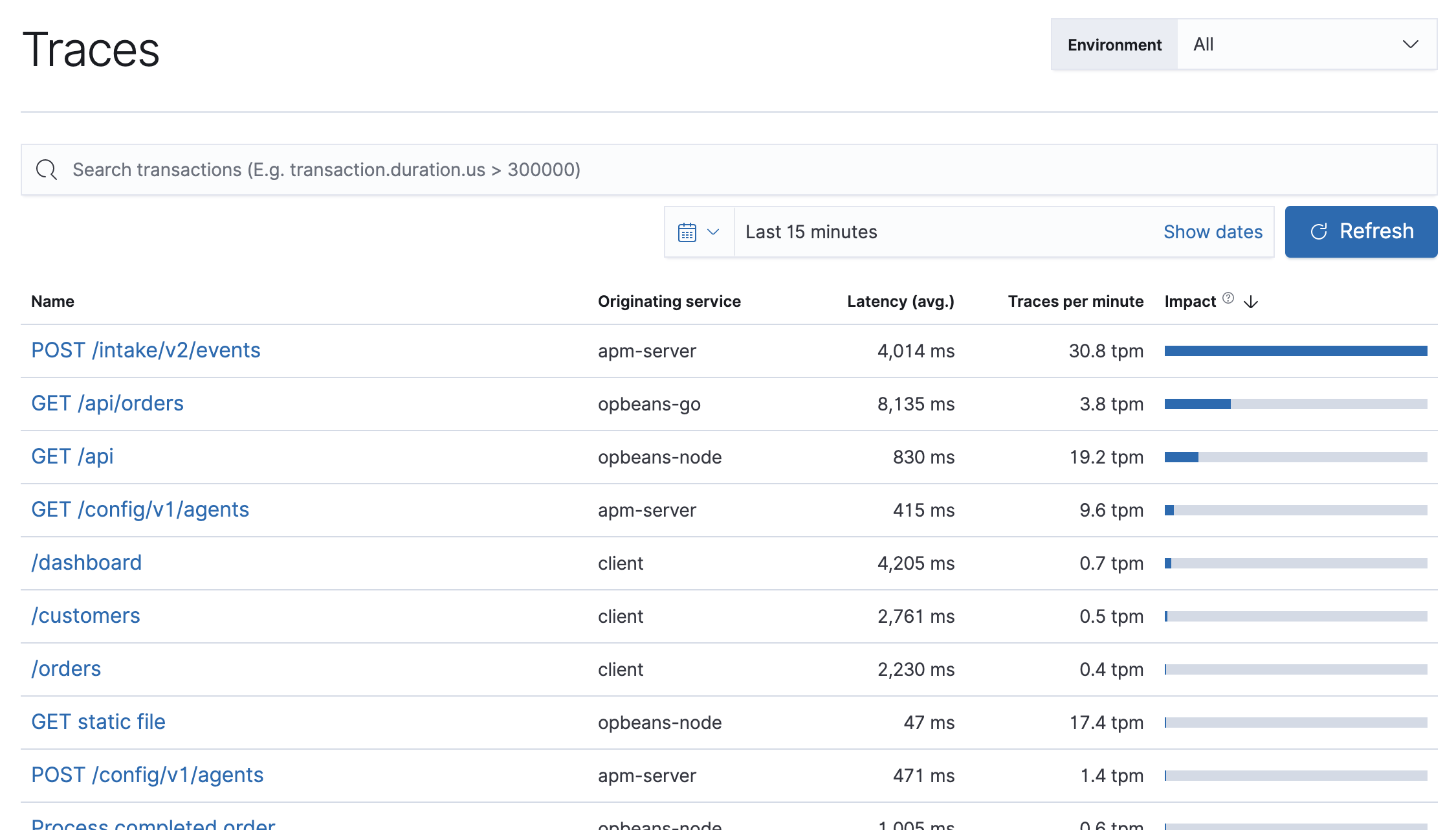**Detailed Descriptive Caption:**

This screenshot captures the 'Traces' section of a web interface, which appears to be part of an application performance monitoring tool. Dominating the upper left corner is the title "Traces." Directly below the title is a search bar with placeholder text that reads "Search Transactions." Adjacent to this, there are filter and refresh options to refine or update the displayed information.

To the right of the search bar, a drop-down menu allows users to select a time range for the displayed data, currently set to "Last 15 minutes." Next to this selector, there is a "Show Dates" link and an additional refresh button for quick data refreshes.

In the top right corner, there's a drop-down menu labeled "Environment," which is set to "All." This allows the user to filter traces by different application environments.

The primary content of the interface features a detailed table listing various trace transactions. The table includes the following columns: Name, Originating Service, Latency, Traces Per Minute (TPM), and Impact.

Each row in the table corresponds to a different transaction, providing comprehensive details. For instance:
- One row lists a POST request to "/intake/v2/elements" originating from the "APM Order" service. This transaction has a latency of 4014 milliseconds, 30.8 TPM, and a high impact indicated by a long blue bar. 
- Another row displays a GET request to "/api/orders" with a significantly higher latency of 8135 milliseconds, a much lower TPM of 3.8, and a shorter blue impact bar, roughly one-fourth the length of the previous example.
- Additional rows list transactions such as "config/v1/agents," "dashboard/customers/orders," "GET static file," and "POST config/v1/agents," each with varying latencies, TPMs, and impact bars.
- Notably, the final transaction in the list, labeled "process completed order," is partially cut off at the bottom of the image.

The combination of these elements provides a clear and detailed overview of the performance and impact of various transactions within the monitored application.